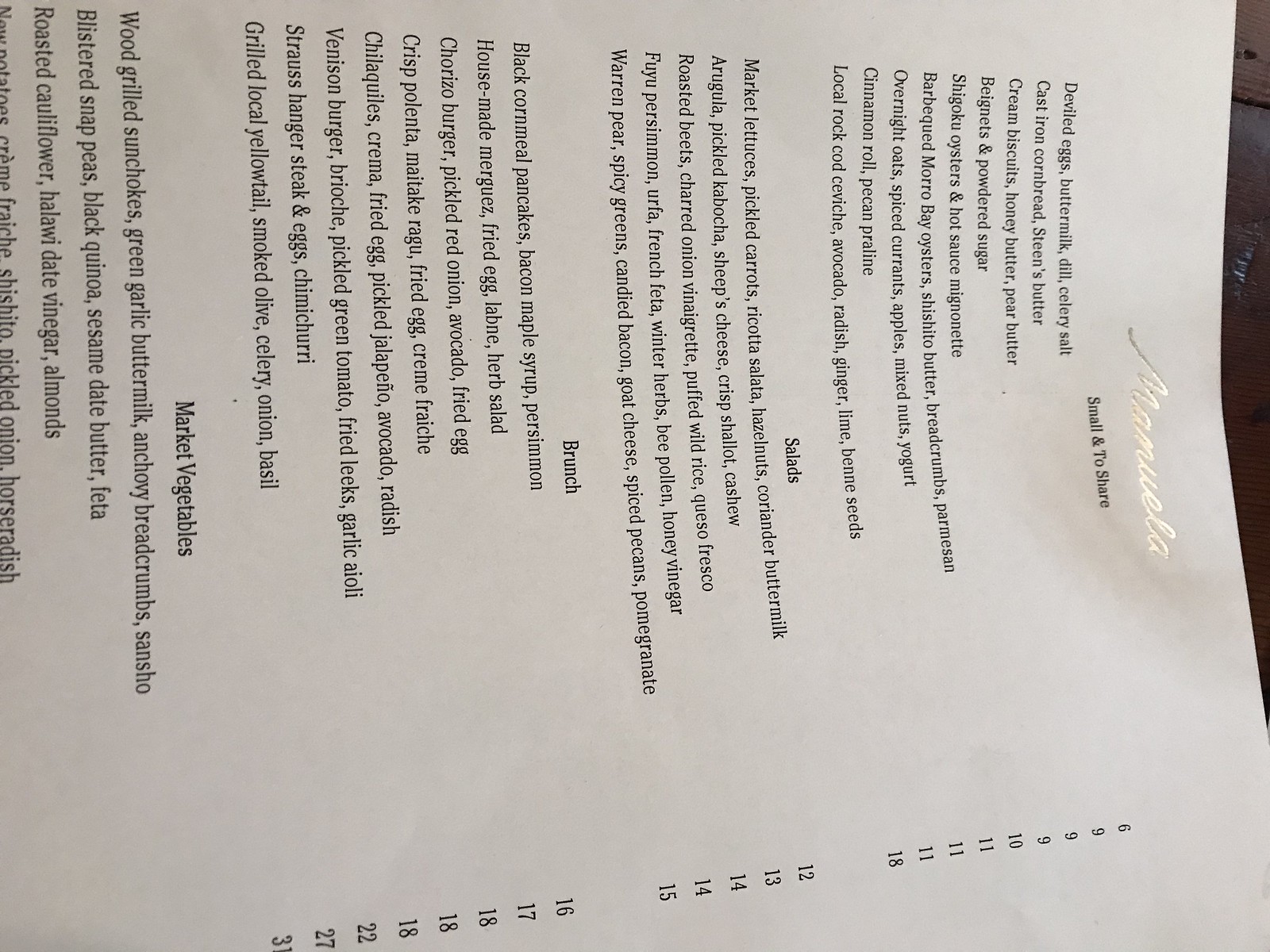This photograph features a sheet of paper positioned sideways, with its orientation having the top part towards the right side of the image. The paper itself is white, sporting a distinctively metallic cursive inscription at its top-right corner that reads "Mar-ma-mula." Just beneath this, there is small text indicating "small and to share."

The layout of the document includes multiple text blocks, aligned predominantly on what becomes the left side of the page due to the sideways presentation. These blocks are interspersed with various category headings. On the right side of the document, visible at the bottom of the image, there are numbered items correlating with the text blocks opposite them on the left.

The background reveals wooden panels on the right side of the image, adding texture to the scene. A notable feature of the paper is a visible crease located at the top-right, adding to the document's character. The overall appearance suggests that this sheet might be a table of contents, likely for a book or similar publication.